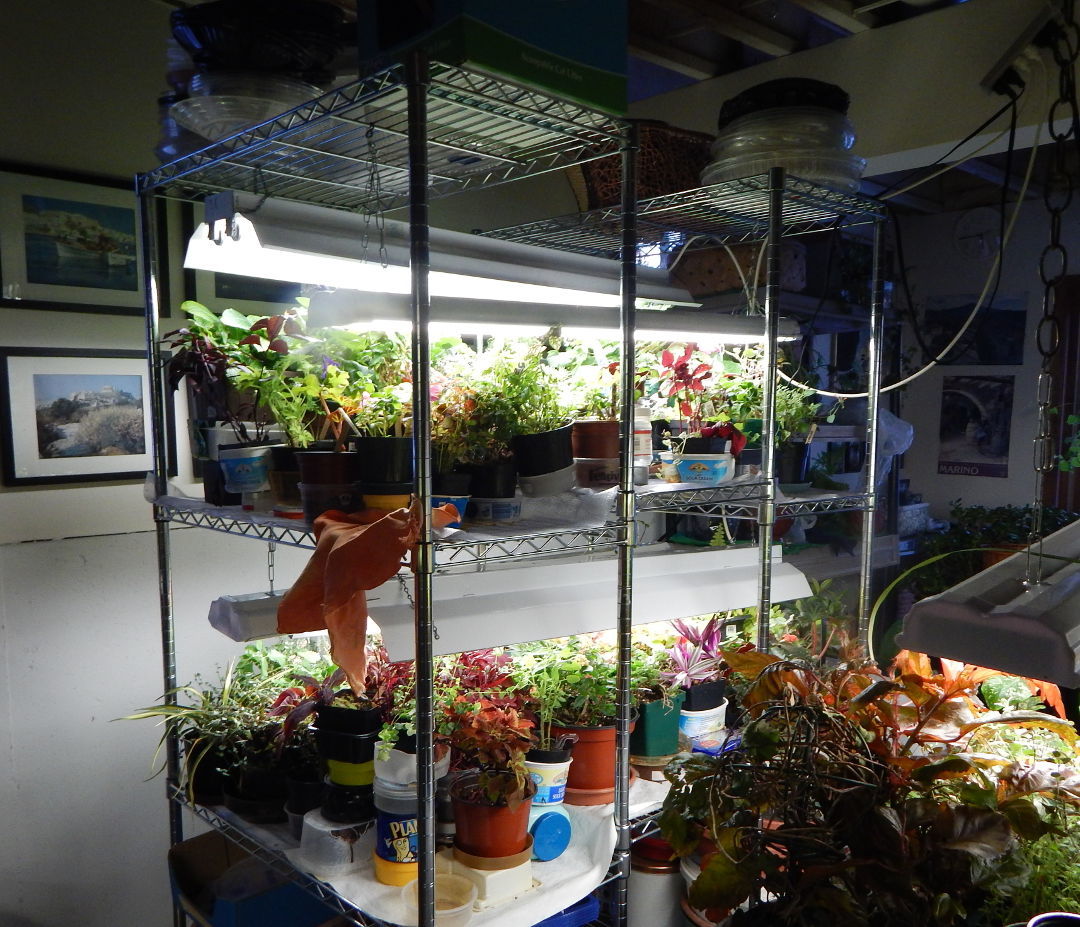This image depicts an indoor garden room, likely part of someone's home. The room features multiple silver shelving units filled with a diverse array of small plants. Each shelf is equipped with bright grow lights to nourish the plants. The bottom shelves hold plants sprouting in various colors—green, red, and purple—placed in an assortment of containers, including round pots, peanut jars, cottage cheese cartons, and butter tubs. Above these shelves, additional plants benefit from the light of a hanging fluorescent fixture, secured by chains. The background of the room reveals a white wall adorned with several framed photographs in black frames, showcasing landscape and water scenes. There are more plants situated below these pictures on the far wall. Although the room appears dark overall, the strategic placement of grow lights ensures the plants receive the necessary illumination to thrive. Some of the ceiling appears to be open, revealing rafters above the setup.